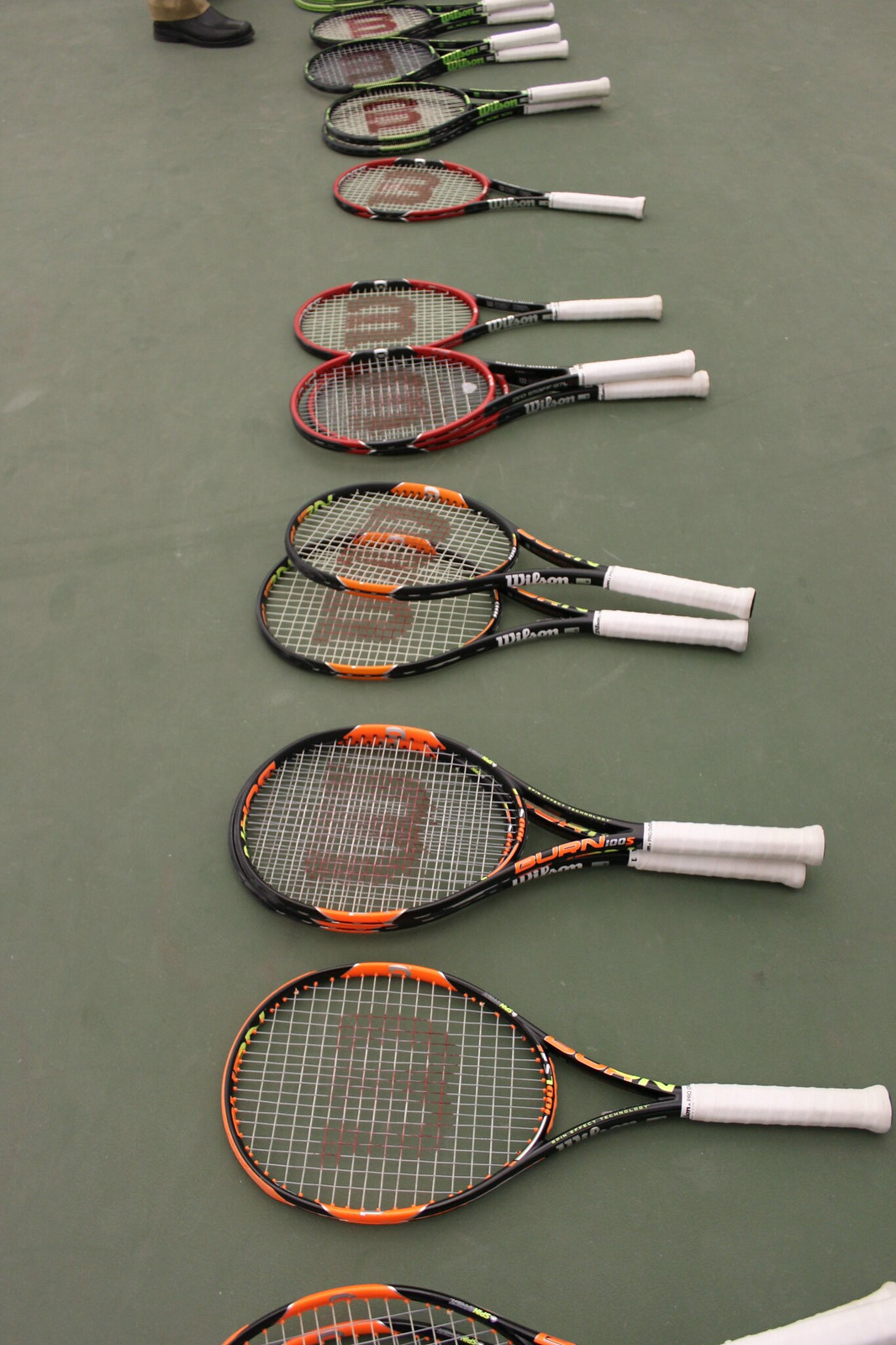The amateur photo, taken in a vertical rectangle format, showcases a close-up of several Wilson tennis rackets intricately arranged on a gray pavement. At the forefront, the rackets, identifiable by the prominent "W" emblem at the center of their white mesh, have orange and black frames with white handles. As the eye moves upward, the arrangement reveals a neat progression: the middle group features rackets with red outlines, and the farthest set in the background displays black and green frames. Some rackets lie side by side, while others are stacked in twos, forming five pairs. At the top left of the image, partly cropped out, is a black boot or shoe with a hint of a khaki brown pant leg. There are no additional texts or markings in the image.